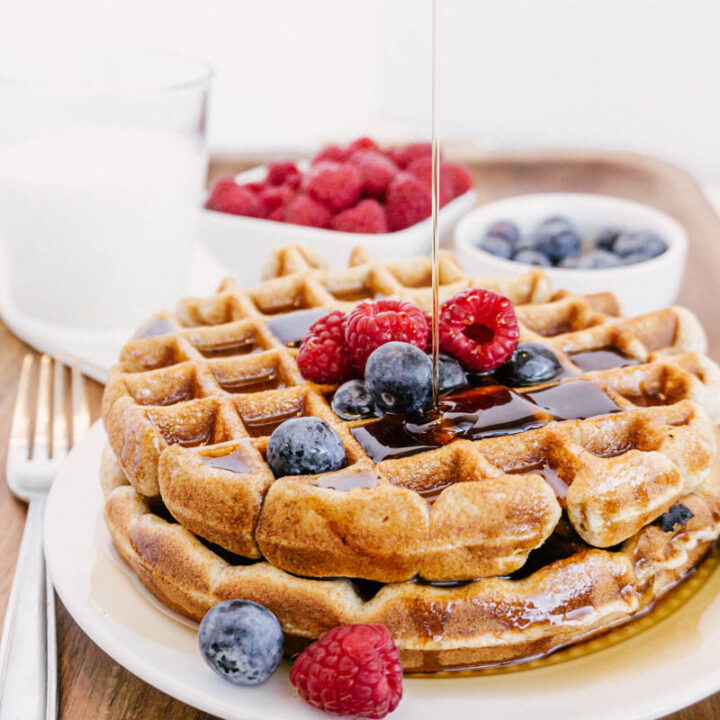This photograph captures a delightful breakfast scene set on a rustic wooden tabletop. At the forefront sits a white, round plate holding two golden-brown waffles. These waffles are elegantly topped with a scattering of fresh blueberries and vibrant red raspberries, with a single blueberry and raspberry adorning the edge of the plate. A thin stream of rich, dark maple syrup is seen being drizzled over the waffles, adding a glossy finish to the appetizing stack.

To the left of the plate, a silver fork rests on the wooden surface, ready for use. In the background, slightly out of focus, there is a glass filled with a clear liquid, likely water, and two small white bowls. One bowl on the left contains raspberries, while the bowl on the right holds blueberries. The background is a soft, out-of-focus white, possibly a wall, bathed in natural, indirect light that offers a cozy, inviting ambiance to the setup.